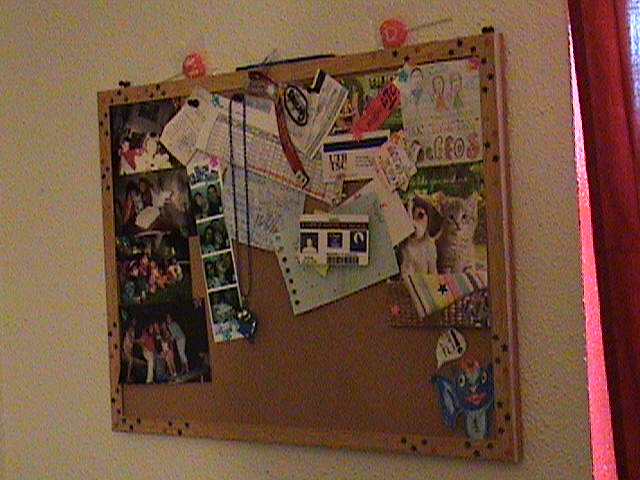This grainy, somewhat out-of-focus snapshot captures a cork bulletin board mounted on a textured, tan stucco wall. The natural wooden frame of the cork board is adorned with colorful polka dots, star stickers, and numerous thumbtacks, particularly in the corners. The board is a collage of personal memorabilia, featuring an eclectic mix of larger and smaller photographs, including images of a cat and a dog. There are also scattered drawings, schedules, receipts, tickets, a card addressed to 'gorgeous,' and a driver's license. A necklace hangs from the left side of the board, and two heart-shaped lollipops are perched at the top. Bright sunlight creates a stark highlight along the right edge, illuminating what appears to be a pink-painted windowsill adjacent to the cork board.